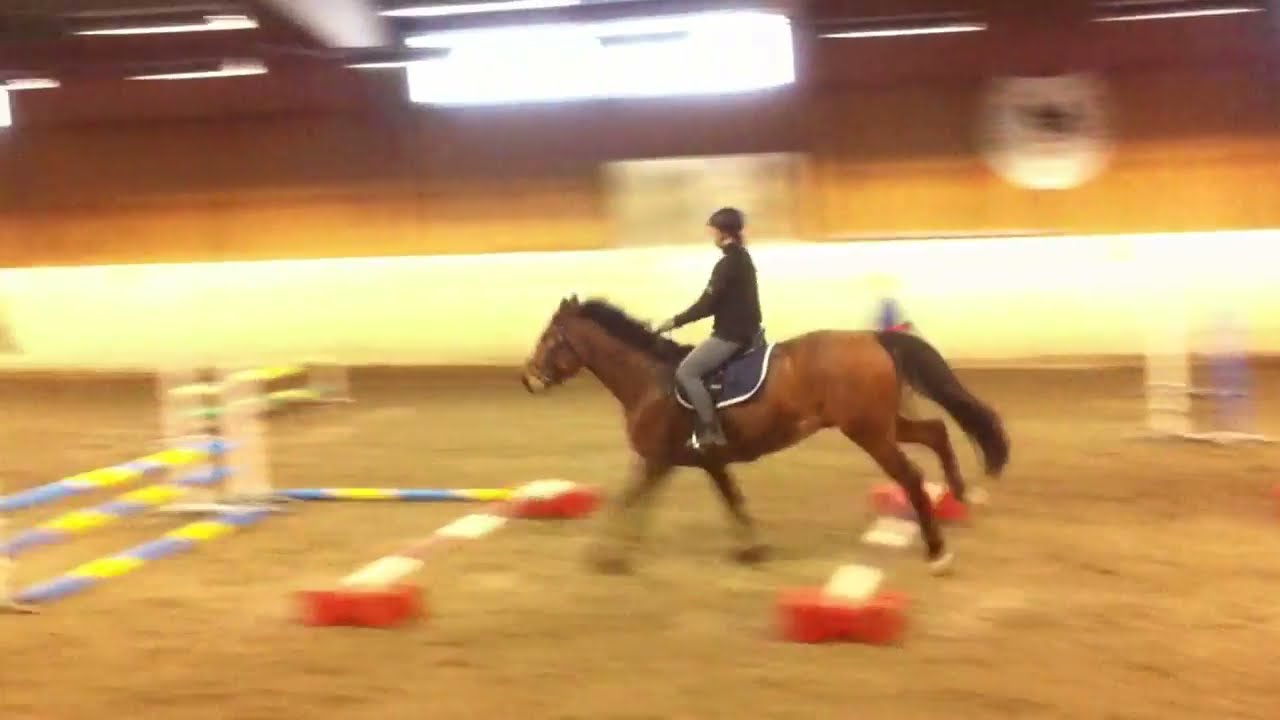In this atmospheric indoor equestrian stadium or training location, captured in a blurred photographic style, a woman outfitted in a black equestrian helmet, a black jacket, and gray pants is seen dynamically riding a large brown horse with a black mane and tail. The powerful horse is captured in mid-leap, clearing a set of red, blue, yellow, and white hurdles, with three bars still in place and one bar fallen to the ground. They are heading toward another hurdle in this challenging jumping event. The arena's dirt floor is a mix of brown and light brown hues, while the backdrop features a mix of brown and white walls and faint fluorescent lighting. A broad window in the background allows additional light to illuminate the scene. Adding to the competitive ambiance, the rider is seated on a black saddle with a blue cloth underneath. Despite the blur, the intensity of the moment is palpable, reflecting the skill and coordination between horse and rider.